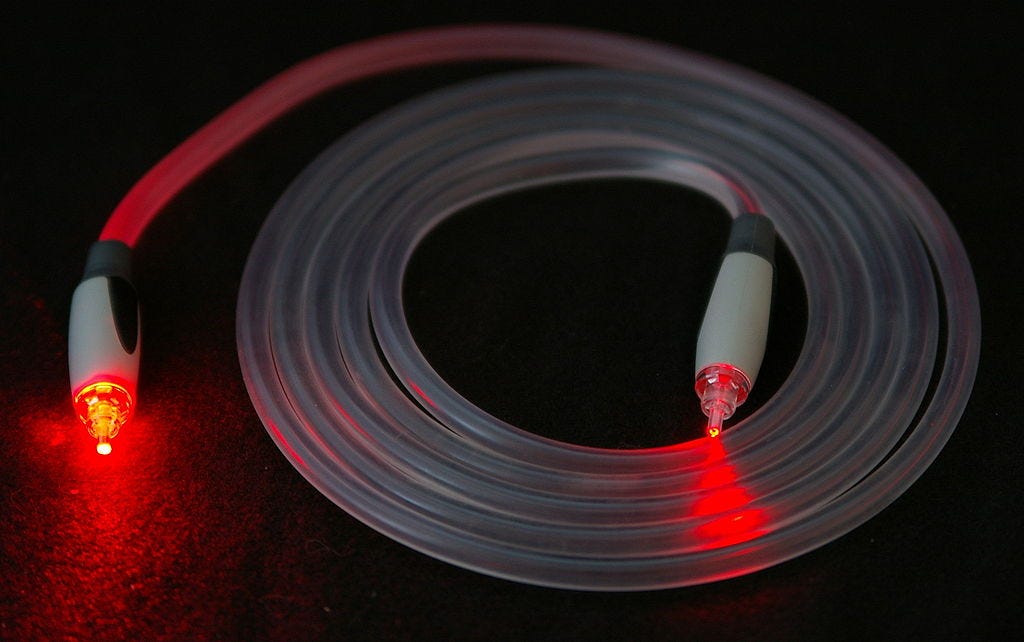The image features a coiled cable set against a black background. The cable appears to be made of a clear, translucent plastic material, looping around six times. Each end of the cable has identical black and light gray tips, with no male or female differentiation, making them unconnectable to each other. Both ends emit a bright red laser light, vividly illuminating parts of the dark scene. The cable is positioned on what seems like carpet flooring, inferred from the light's reflection on the ground. The end connectors consist of black rubber with gray plastic components that lead to clear sections from which the red lights shine. Overall, the photograph captures a mysterious cable, possibly fiber optic, glowing faintly within the coils and prominently at both tips, creating an enigmatic and striking visual effect in a dimly lit room.